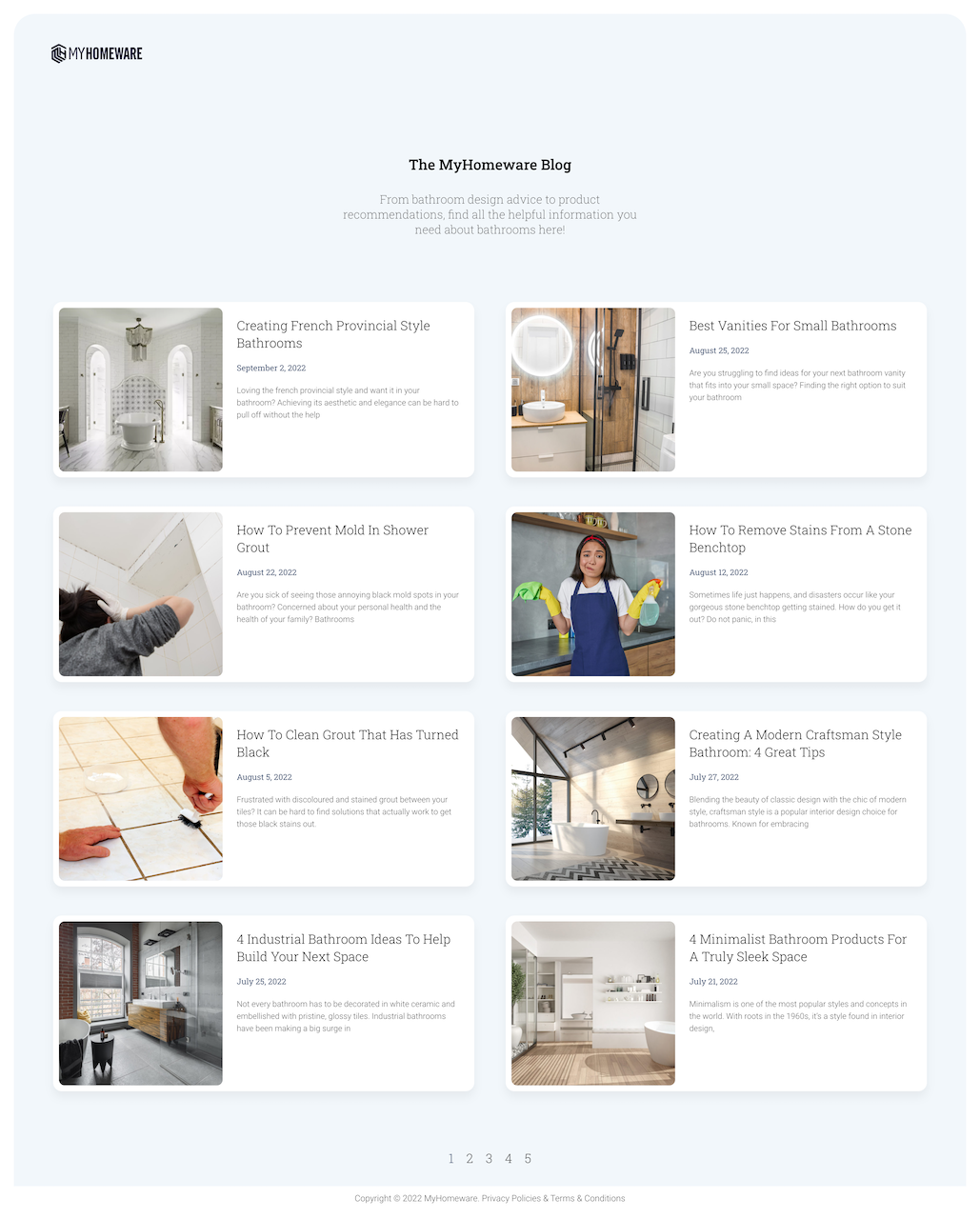This image is a screenshot of the homepage of a blog titled "My Homeware Blog," with "My Homeware" written as one word and both the "M" and "H" capitalized. The page features a light bluish-gray background and displays summaries for eight blog entries arranged in two columns of four. Each summary consists of a thumbnail photograph on the left, accompanied by the title, date, and a brief synopsis on the right.

In the upper left-hand corner, the site's name, "My Homeware," is prominently displayed alongside its logo. Centered at the top, the header reads "My Homeware Blog," followed by a brief description, though the small text makes it difficult to read.

The blog entry thumbnails showcase various home-related themes. One image features a woman in a blue apron, white t-shirt, and cleaning gloves making a shrug with an exaggerated smirk. Another image shows a bathroom with a lighted mirror, while a separate bathroom scene highlights a freestanding tub and large arched windows. Additionally, there is a photograph of someone cleaning dirty grout on tile work. 

At the very bottom of the page, pagination numbers from 1 to 5 indicate that there are at least five other pages of blog entries available.